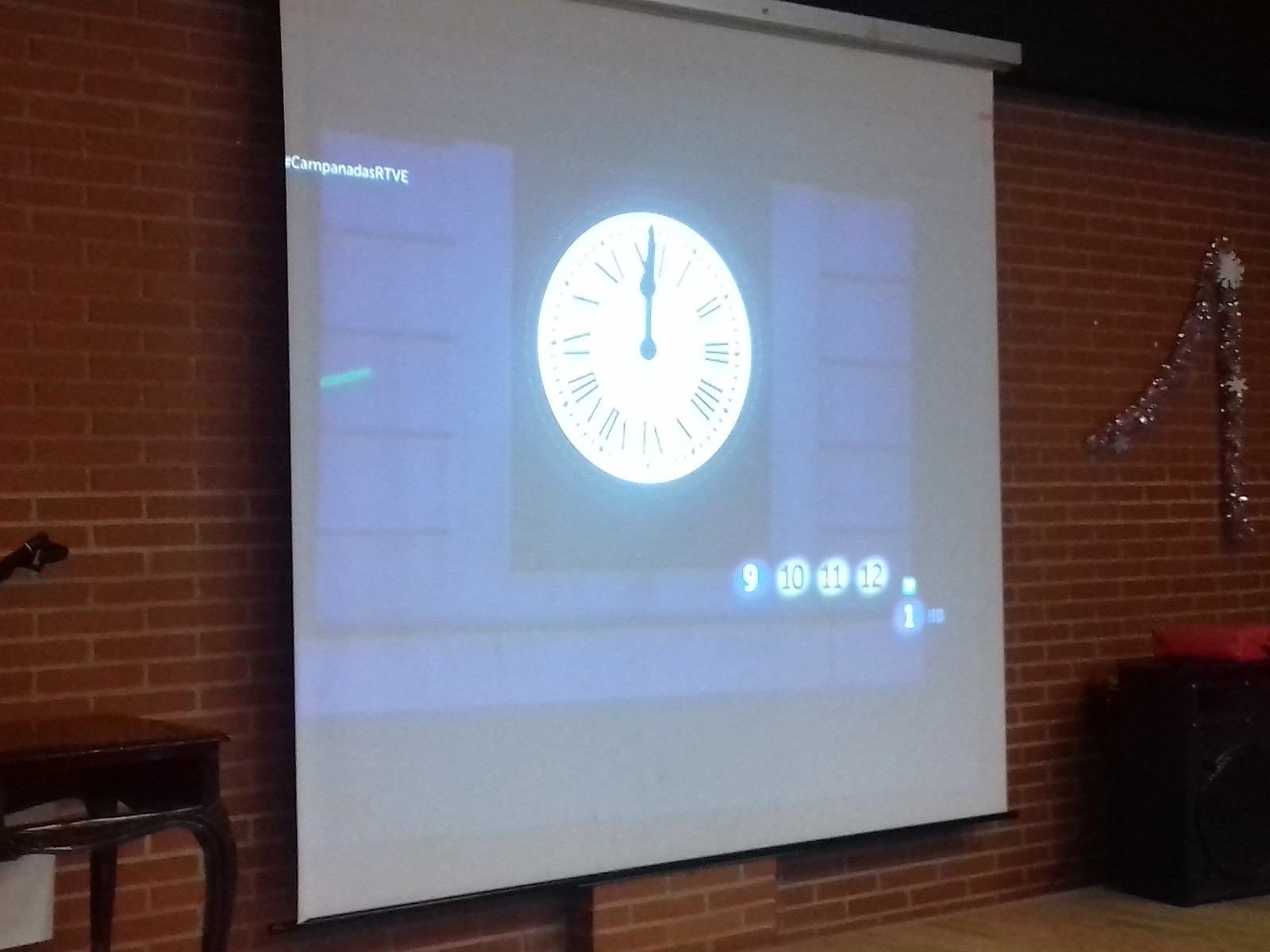In the image, we see a projection screen displaying the face of an old-fashioned clock with Roman numerals. The clock face is clearly projected, indicating that it is part of a visual display rather than an actual clock. There is a watermark on the projection that reads "Camp In Dust RTV VE," along with an accompanying hashtag. The background features a straightforward brick wall adorned with a few decorative elements, such as ornamental streamers. Below the projection screen, there appears to be an amplifier placed against the wall.